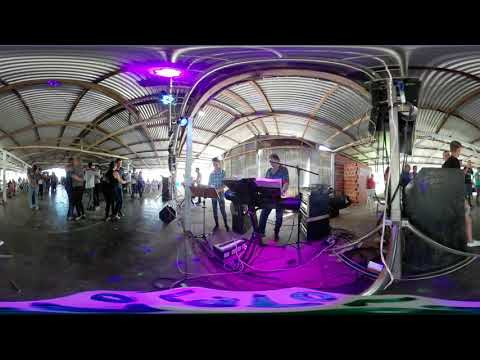The image captures a visually appealing scene inside a large metal building or potentially a tent-like structure with a metal canopy, featuring what appears to be a band or performers on a stage. The roof showcases three arches with a wood-like framework crossing horizontally and vertically. A prominent white light surrounded by a purplish glare casts a captivating hue over the scene, with additional stage lights and natural light filtering in from above.

In the foreground, at the center of the image, a performer stands at a keyboard with a music stand and sheet music in front of him. Another individual stands nearby, positioned at a music stand. Several speakers and electrical equipment are set up around them, emphasizing the importance of the central performance.

Towards the left side of the image, a crowd of people gathers, intently watching the performers. There is an easel and platforms positioned in front of the musicians, suggesting a structured setup for the performance. The floor beneath them exhibits a purple haze, possibly from the stage lights or reflections, along with distorted blue letters or numbers, hinting at some form of banner or signage.

The backdrop includes elements of red brick walls, adding a touch of contrast to the metallic and vibrant light setting. With three separate frames creating a panoramic effect, the image captures both the intensity of the performance and the dynamic atmosphere of the audience, seamlessly blending the vivid purple illumination and the natural and artificial lights of the stage environment.

Overall, the combined details create a rich, immersive scene of a musical event, highlighting the structural and atmospheric elements of the venue and the engaged crowd.